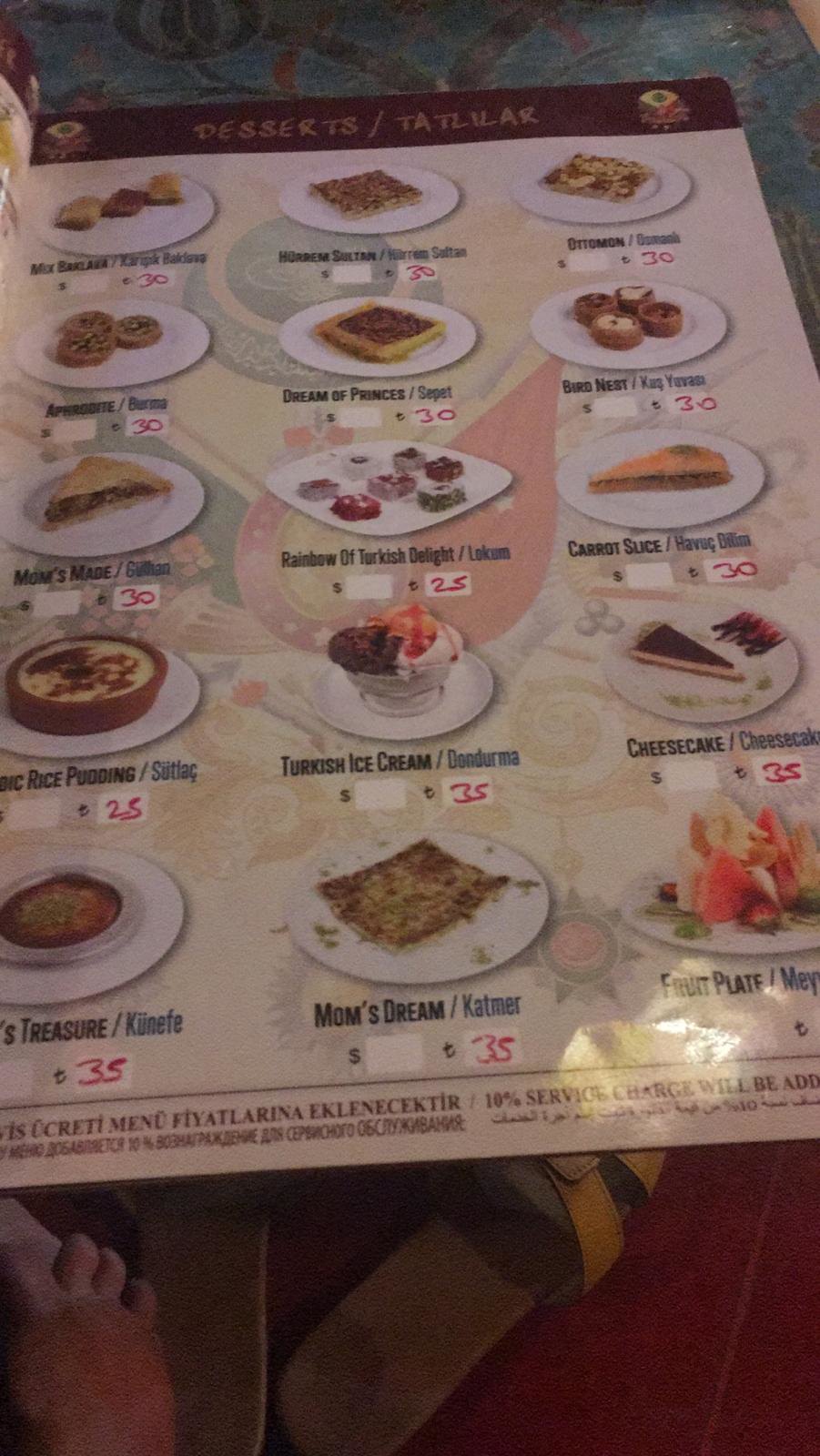The photograph depicts a restaurant menu, elegantly framed against a vivid backdrop. At the top, the background showcases a tranquil blue hue adorned with lush green plant leaves. The lower portion of the image contrasts with a vibrant red floor, partially obscured by a yellow and brown sandal revealing three toes of a person’s foot.

The focal point, the menu, prominently features a title “Desserts / Tatliyar” in a bold, red-bordered box set against a white background enhanced with ornate red, green, and yellow patterns. The menu lists an array of enticing dessert options, intricately named and priced as follows:  
- Mix Baklava: $30  
- Horim: $30  
- Sultim: $30  
- Ottoman: $30  
- Aphrodite: $30  
- Dream of Princes: $30  
- Bird Nest: $25  
- Mom’s Maid: $30  
- Rainbow of Turkish Delight: $25  
- Carrot Slice: $35  
- Rice Pudding: $35  
- Turkish Ice Cream: $35  
- Cheesecake: $35  
- Treasure: $35  

The pricing for the "Fruit Plate" is unfortunately not visible as it is cut off in the image.